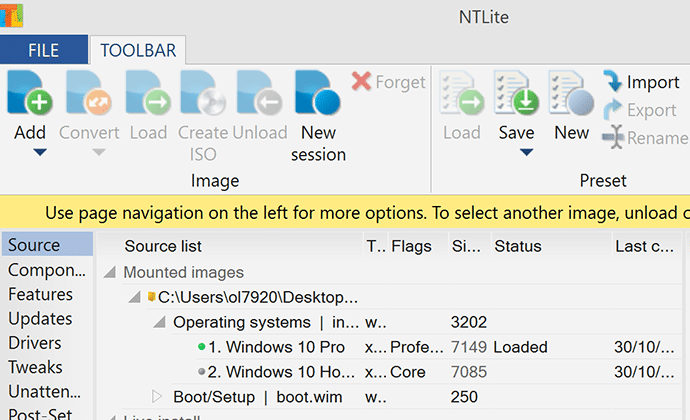This image captures the user interface of a computer application, which appears to be an ISO or CD burning software. The interface features a light gray background with a darker gray top portion. In the upper left corner is a colorful square icon with an orange 'T', and possibly blue, yellow, and orange elements forming an 'I' and an 'L'. To the right, the title "NT Lite" is displayed.

At the uppermost section, there are two tabs: 'File' (in white letters on a blue background) and 'Toolbar' (in blue letters on a gray background), with 'Toolbar' currently selected. Below 'Toolbar,' a series of function icons are listed horizontally: Add, Convert, Load, Create ISO Image, Unload, New Session, and Forget (marked with an X). To the right are additional functions grouped vertically: Load, Save, New, Import, Export, and Rename.

Below these toolbar options, a yellow-highlighted message reads, "Use page navigation on the left for more options. To select another image, unload," with the remainder of the text cut off. The lower portion of the interface contains two main columns. On the left, it lists: Source, Component, Features, Updates, Drivers, Tweaks, Unattend, and Post Setup. The right column displays a source list and status information labeled "tfraxed."

Additionally, a file explorer window is visible at the bottom, with a navigation path indicating the destination C:\Users\OI7920\Desktop. Overall, the interface is designed for managing ISO images and possibly other file-related tasks.